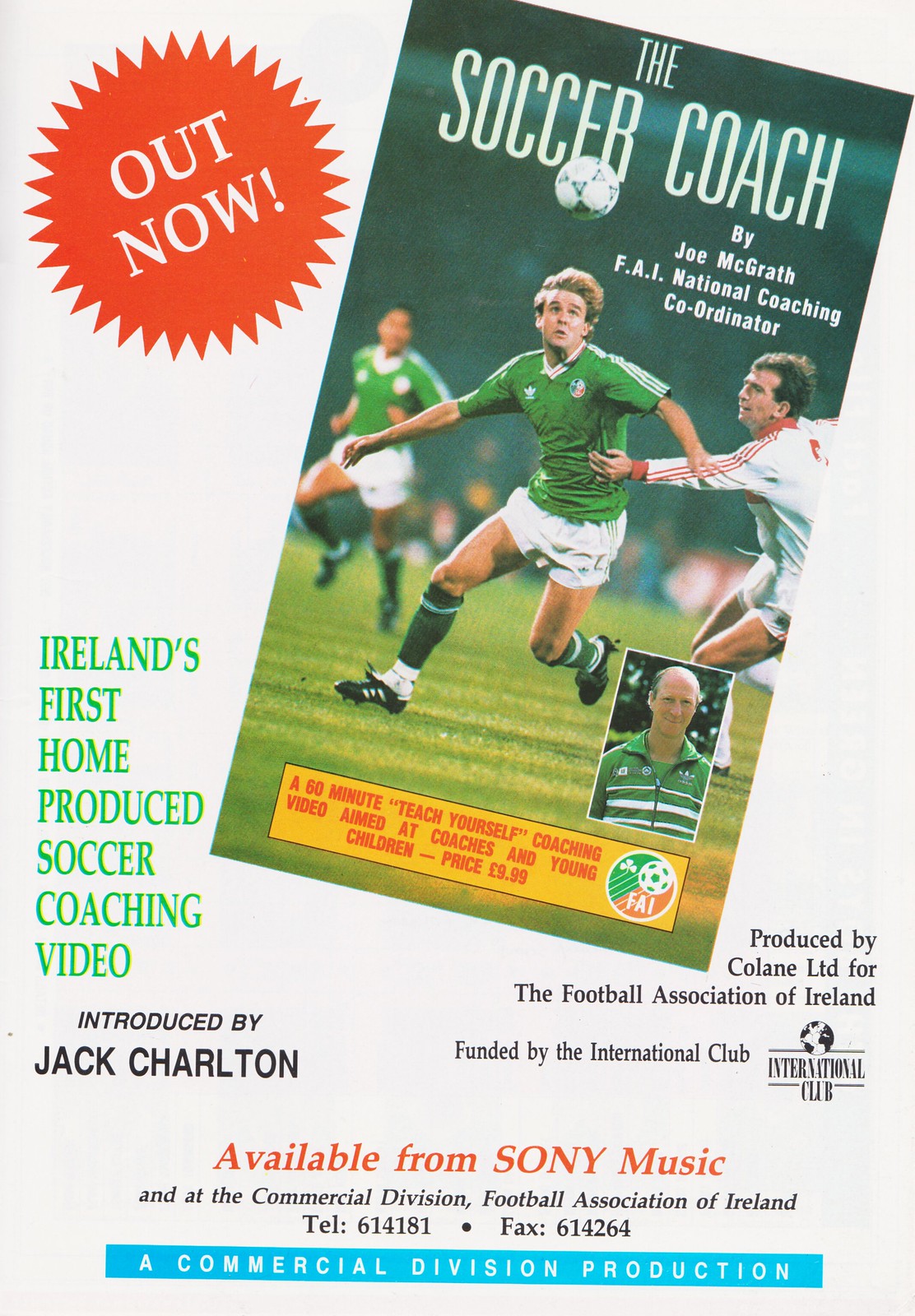The image is an advertisement for a soccer coaching video titled "The Soccer Coach" by Joe McGrath, the National Coaching Coordinator for FAOI. The cover of the video features a dynamic photograph of two players competing for a soccer ball, one wearing a red and green jersey and the other in a white jersey. Prominently displayed on the cover is a starburst that announces "Out Now," along with text indicating that this is Ireland's first home-produced soccer coaching video, introduced by Jack Charlton. The video's description highlights it as a 60-minute, teach-yourself coaching resource aimed at coaches and young children. At the bottom of the cover, it states that the video is available from Sony Music and provides both a telephone number and a fax number for contact. The design incorporates a variety of colors, including red, white, dark green, light green, brown, light blue, and teal, with black and white text. The image appears to be taken outdoors, capturing a real-time shot during a game.